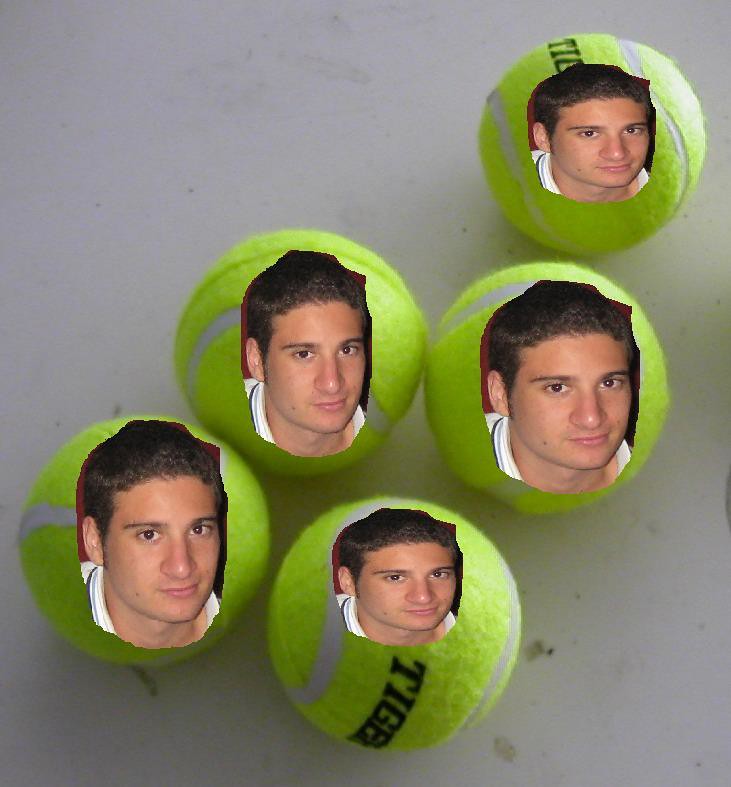The image is a color photographic montage featuring five tennis balls placed on a white table with a slate gray background. These yellow-green tennis balls, reminiscent of dog toys due to their lower quality, have broad white lines and one bears a partially visible black logo, seemingly spelling out "tiger." Each tennis ball displays the digitally superimposed face of a young man with brown hair, combed back, and long sideburns. The man, wearing a white collared shirt, sports a neutral expression, with his bushy eyebrows and direct gaze adding to his intense look. The faces are manipulated to vary in size and proportion across the tennis balls, creating an eerie yet artistic composition. The balls are arranged with one near the top right, two side-by-side in the middle, and another two side-by-side closer to the bottom left of the image.